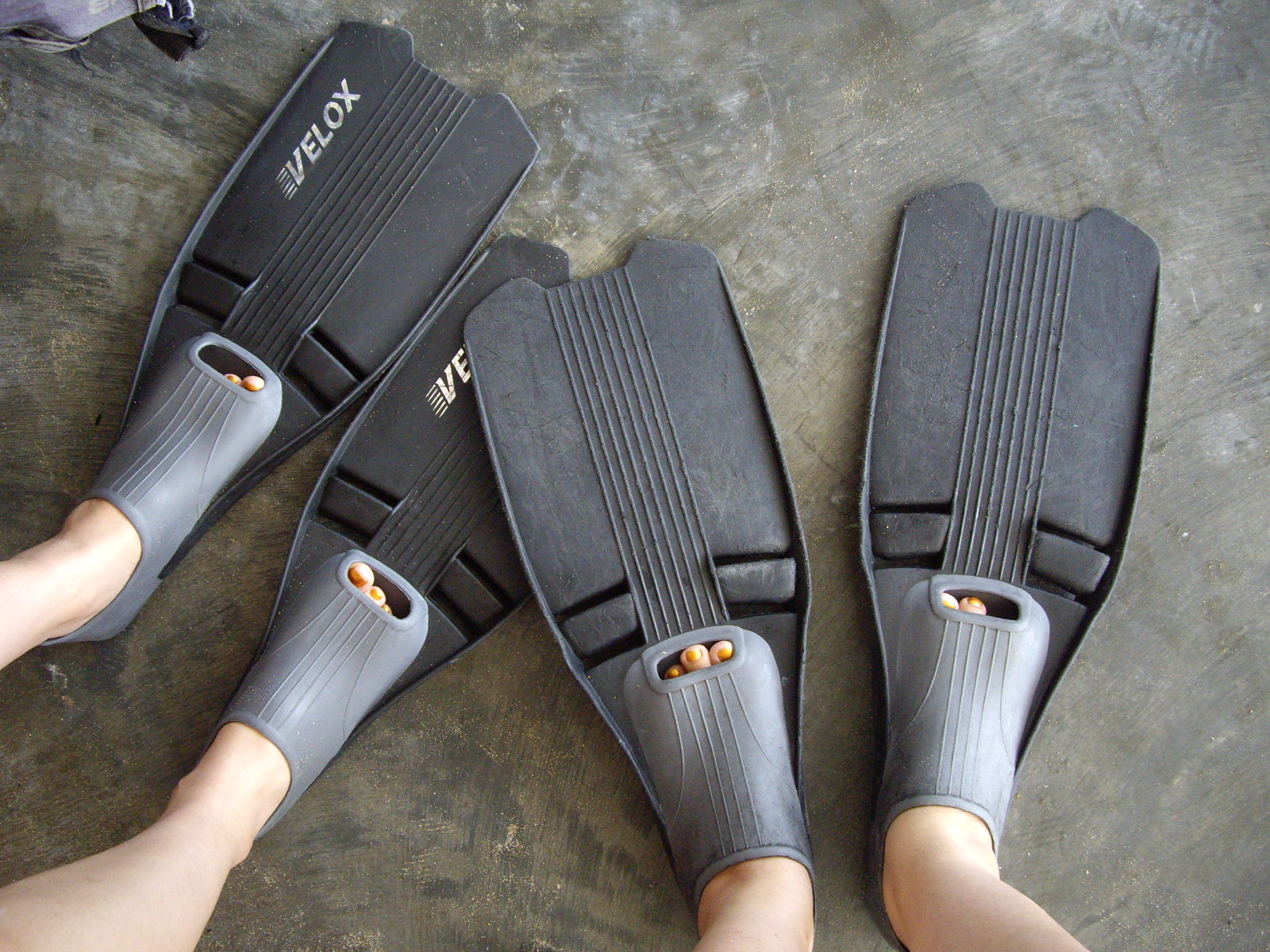The photograph captures the feet of two individuals, both wearing black and grey swimming flippers designed for diving or snorkeling. The flippers have a grey section enveloping the feet, with visible toes peeking through small openings at the top; the toenails are painted a metallic orange. The larger parts of the flippers are black, featuring the brand name "Velox" in white text along with central striations. The individuals appear to be female and stand on a well-worn concrete floor that ranges in color from light to dark grey, revealing brush strokes and a weathered surface. In the top left corner of the image, there is an indistinct object.